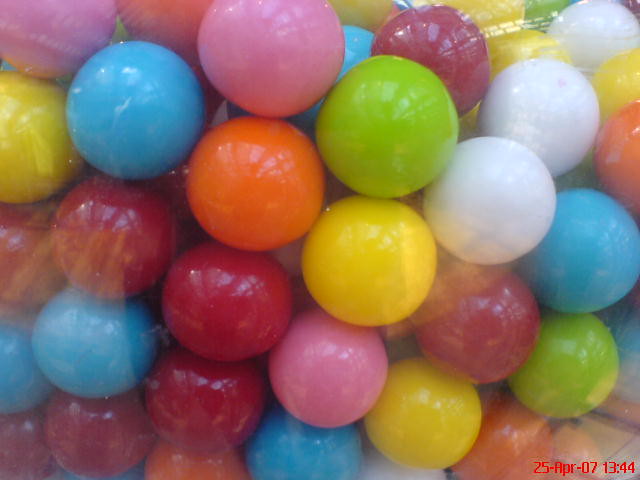This image showcases a collection of brightly colored plastic balls, reminiscent of those found in a children's play zone. The balls, varying in hues of red, light blue, orange, yellow, green, white, maroon, pink, and lime green, are clustered together, creating a vibrant and playful scene. They appear to be made of a shiny plastic material, reflecting light and displaying signs of wear such as gray scratches and denting. The balls are stacked in a somewhat organized manner, viewed at a diagonal angle that gives depth to the photo. In front of the balls, a transparent pane of glass or plastic reveals reflections, possibly of windows. A date and time stamp are visible in red text at the bottom right corner, reading "25 April 07" and "1344."